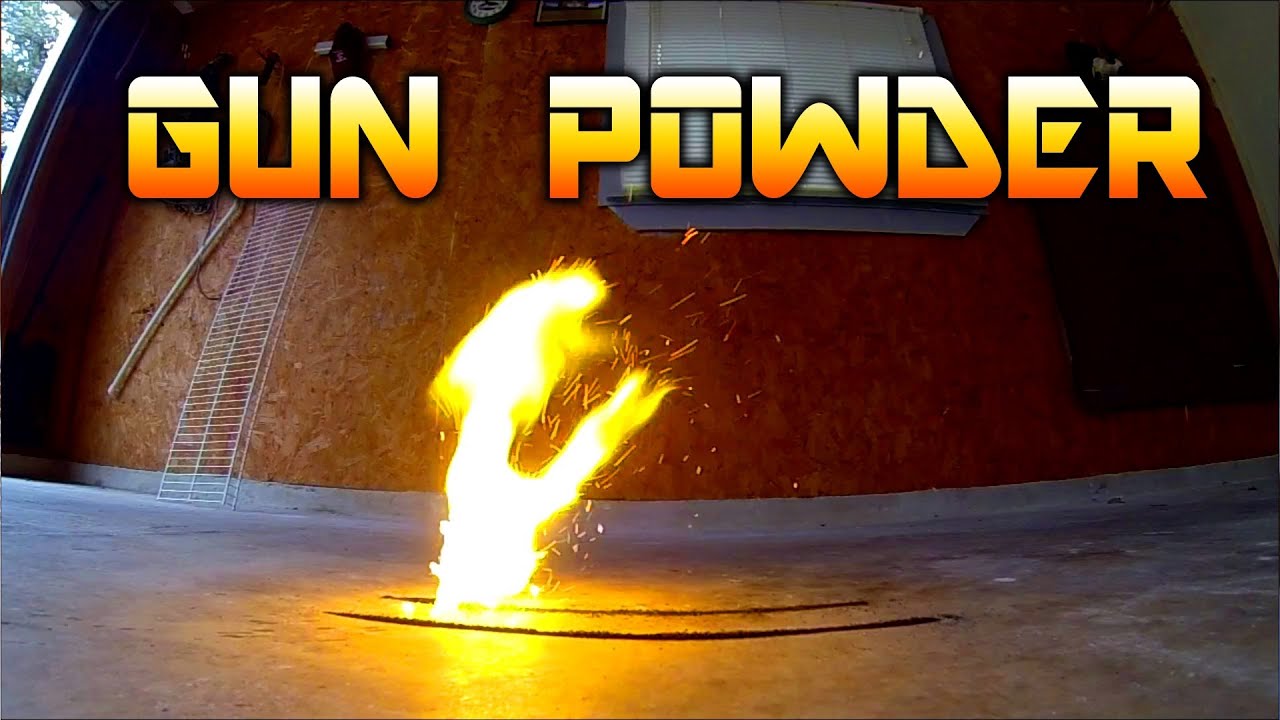The image captures a scene inside a garage with concrete flooring and corkboard-covered walls. A window with blinds is barely visible on the left-hand side. In the upper left corner, part of the garage door is open, revealing a glimpse of trees outside. Dominating the top of the image, large text in a gradient from bright to darker orange reads "GUNPOWDER." 

On the concrete floor, two dark lines of gunpowder are laid out, appearing to be ignited, with visible flames. The flames are predominantly a bright, whitish-orange color, transitioning to yellow at the edges, highlighting the ignition process. In the left corner, a white rack leans against the wall, adding to the setting's makeshift, experimental feel. The image's color palette includes yellows, browns, oranges, grays, and blacks, emphasizing the fiery effect and the industrial environment of the garage.